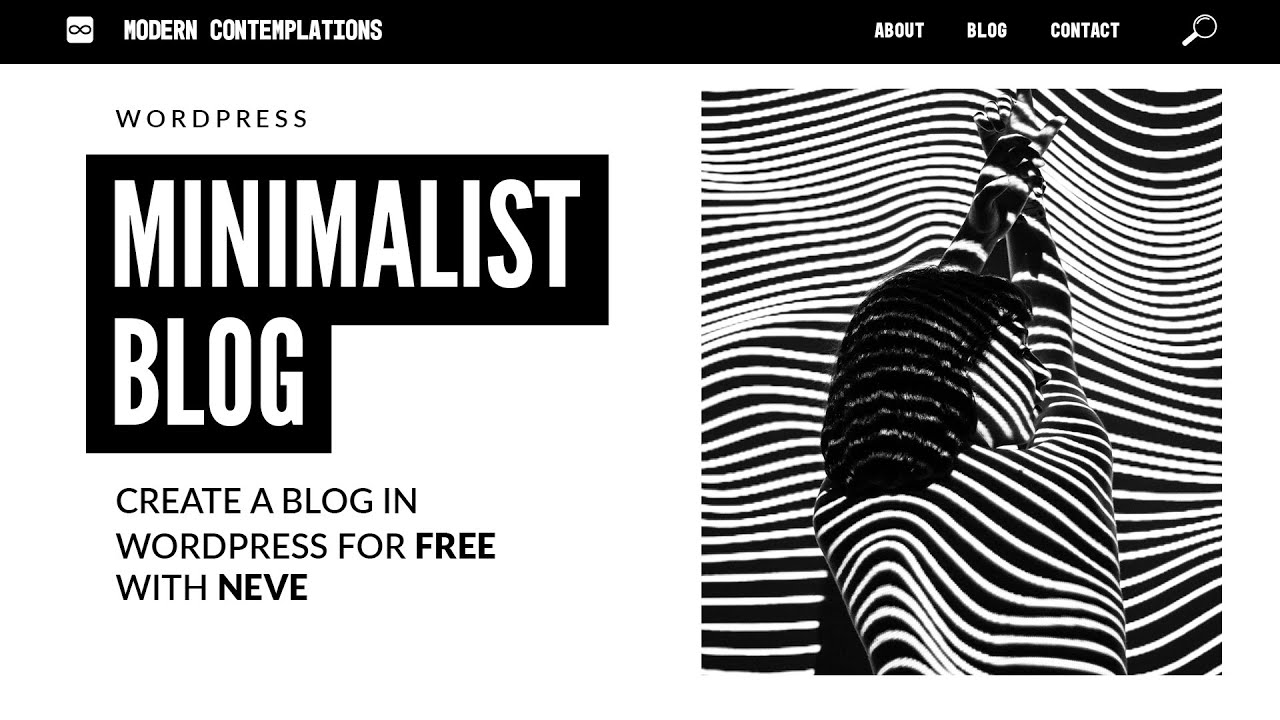This image is a detailed screenshot of a black-and-white web page, square in shape. The page features a prominent black navigation bar at the top, inscribed with white text. Starting from the upper left, the text reads "Modern Contemplations," accompanied by a small logo resembling either an infinity sign or eyeglasses, all set within a white square on a black background. To the right side of the navigation bar are clickable links for 'About,' 'Blog,' 'Contact,' and a magnifying glass icon indicating a search function.

Below the navigation bar, on the left side of the page, the word "WordPress" is displayed in black text against a white background. Beneath this, there is a bold black L-shaped box containing the words "Minimalist Blog" in white capital letters. Directly under this box, black text reads, "Create a blog in WordPress for free with Neve," the latter part emphasized with "Neve" in all caps. 

Dominating the entire right side of the page is a square abstract image. The image, formed by intricate black-and-white stripes, appears to represent the back of a woman. Her black hair and partial face emerge from the intertwined lines, creating a visually captivating and complex pattern reminiscent of zebra stripes.